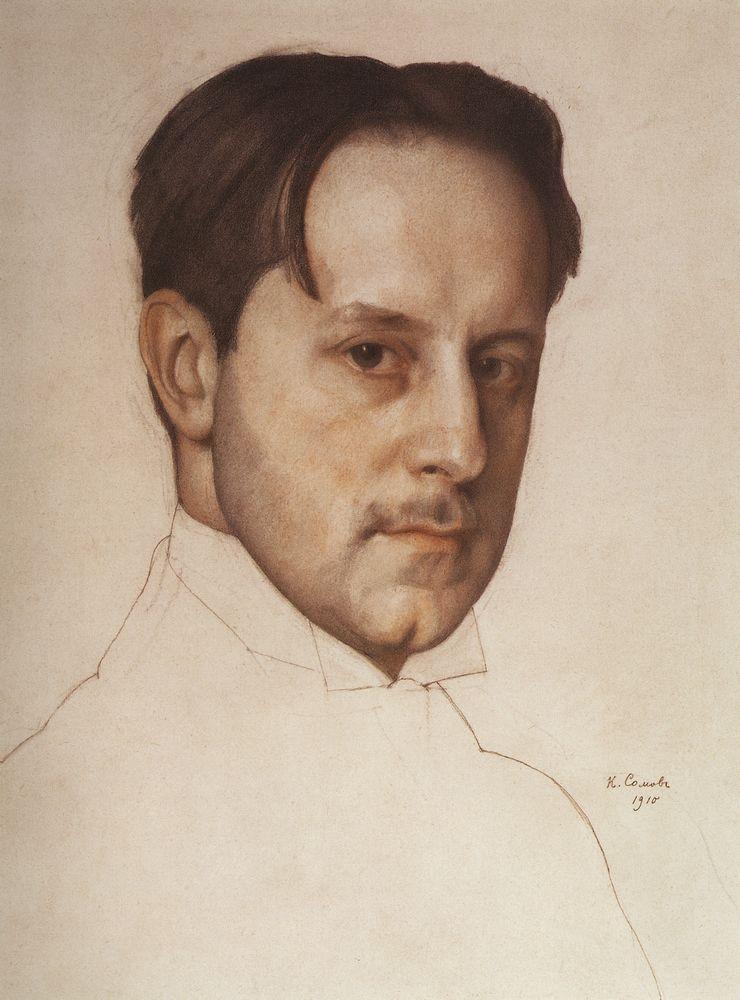The image depicts a detailed and vibrant painting of a man's face, focusing on his features from the neck up, while his body below is merely an unfinished sketch. The man, who has a light skin complexion, short black hair parted in the middle with some bangs over his forehead, brown eyes, and a slight mustache, appears thoughtful as he gazes slightly to the right. His right ear is prominently visible, while his left ear is less so. His face and hair are fully colored, contrasting with the sketch-like outline of his high-necked shirt with open collars, which remains devoid of color.

The background of the image has a warm, stained appearance, resembling light tan or light brown, as if the paper had been soaked in coffee and left to dry. In the bottom right corner, there is a signature and the year "1910," though the exact details are difficult to discern. This combination of detailed facial features and the unfinished body, along with the warm tones of the background, gives the impression of a floating head on a partially completed canvas.